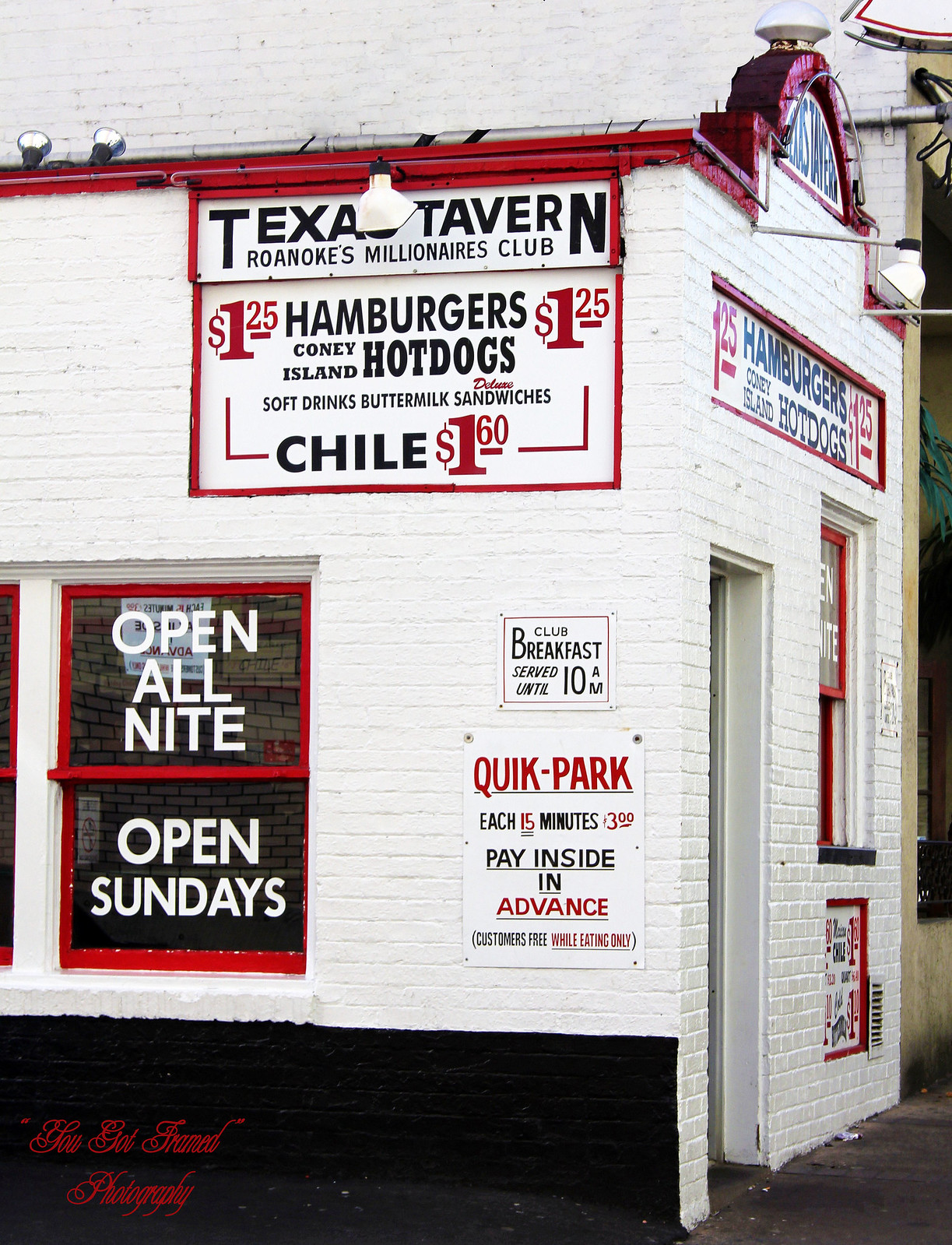This image depicts a quaint, small, white brick building designed to resemble a classic diner or take-out area, prominently painted with red accents and trim. The establishment, identified as Texas Tavern, carries the slogan "Roanoke's Millionaire's Club" and displays a nostalgic charm with its vintage signage. The text on the sidewall advertises various menu items including $1.25 hamburgers, Coney Island hot dogs, soft drinks, buttermilk sandwiches, and chili for $1.60. An additional sign on the left-hand side further promotes club breakfast served until 10 a.m., and emphasizes the convenience with “Quick Park” rates of $3.00 per 15 minutes, reminding customers to pay inside in advance and noting that parking is complimentary while dining. The window towards the bottom left boasts signs declaring the tavern’s round-the-clock service, “Open all night” and “Open Sundays,” enhancing the diner’s inviting and accessible nature. The right side of the building features the main entrance, flanked by additional windows and more signage, consolidating the diner’s nostalgic and welcoming atmosphere. A watermark in the bottom left corner indicates the photograph was taken by "You Got Framed Photography."